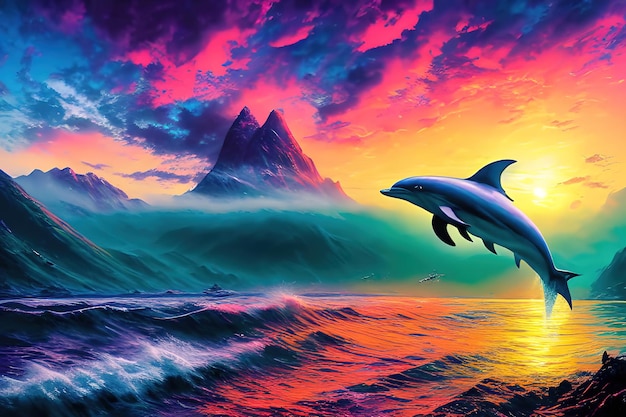In this colorful, computer-generated digital image, a detailed and vibrant scene unfolds. The main focus is a dolphin, predominantly blue on its sides and grayish-blue on its top, with a light gray underbelly. The dolphin is captured mid-leap out of the water, with a total of three fins on its belly, two fins on each side, a skewed-looking triangular tail, and a single prominent dorsal fin on its back. It sports a grim expression, looking straight ahead with a black pupil in a white eye.

The water, depicted with white waves, reflects the myriad colors of the sky, appearing pink and yellow near the dolphin and transitioning to purple and blue as it spreads out. The sky itself is a mix of pink, blue, yellow, white, and purple hues, with the sun—a brilliant yellow—shining from the background to the right of the dolphin. This radiant sun casts a warm glow over the scene, blending and enhancing the colors of the sky and water. Adding to the dynamic landscape, blue mist rolls over a distant mountain range that appears purple and blue. Pink and white clouds float above, completing this visually striking and whimsical portrayal.